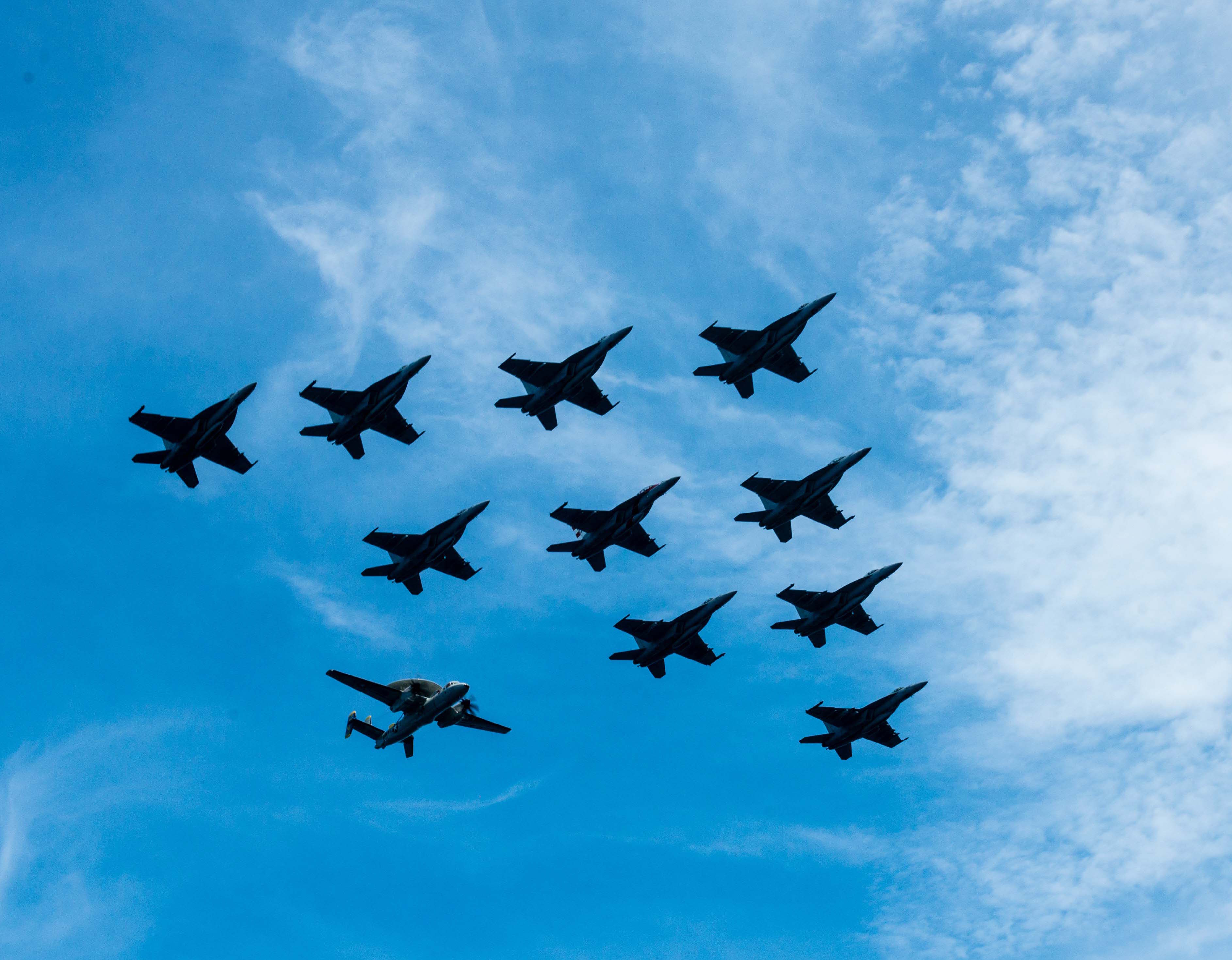In this photo, taken from the ground looking up into the sky, a striking aerial scene unfolds. Against a deep blue sky dotted with light cirrus clouds, ten identical black fighter jets are captured in a precise triangular formation, resembling an arrowhead. Seven jets form the tip, while three more are centered directly behind. Trailing this impressive V-shaped formation is a distinct aircraft with straight wings and a radar dome, likely an AWACS plane, emphasizing its role as a different type of plane among the sleek, swept-wing jets. The photograph, taken during what appears to be an aerial show, magnificently captures the uniform precision and power of these military aircraft in flight.